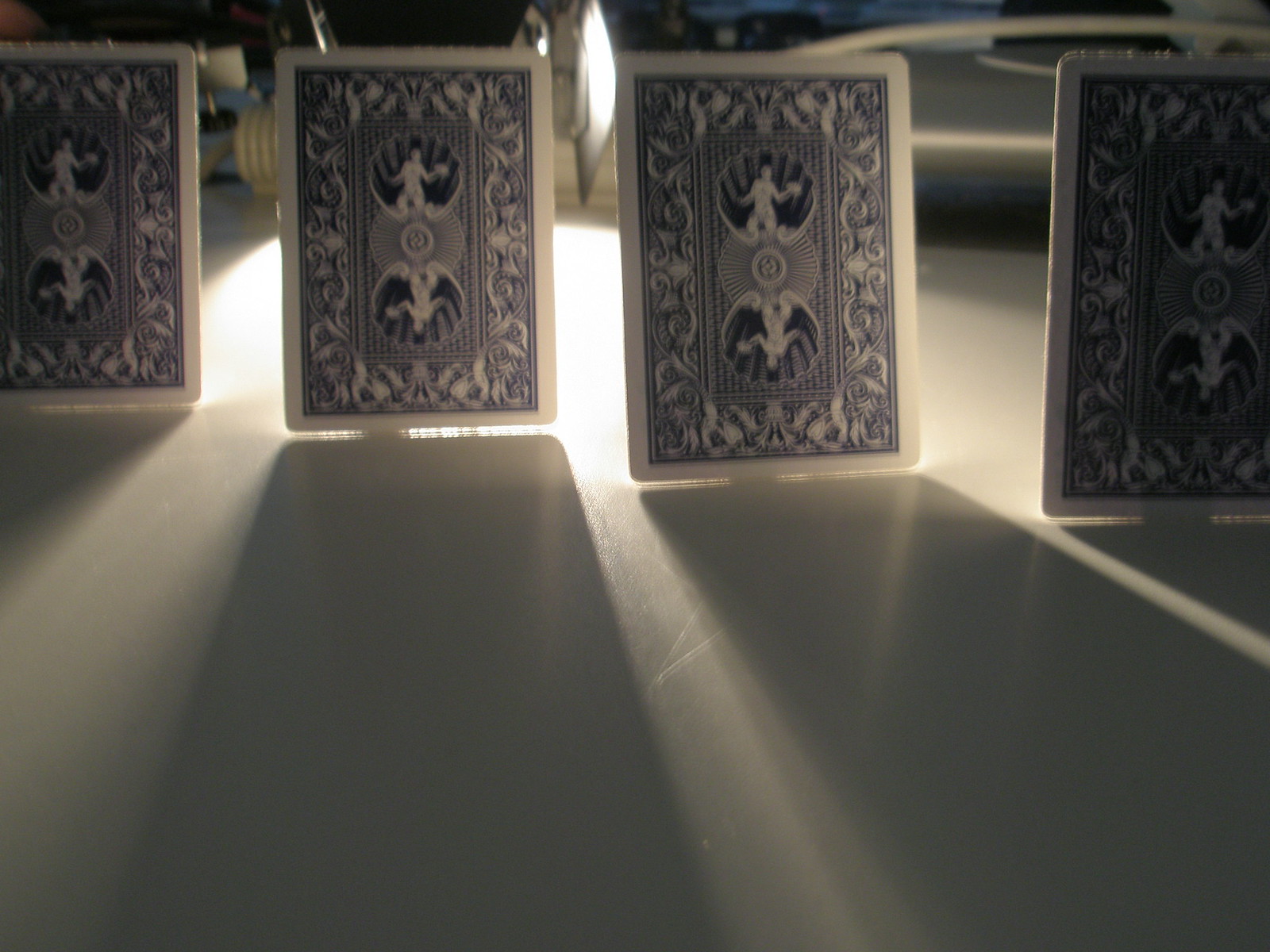This photograph, brightly backlit, depicts a low-angle view of a white, smooth surface, possibly a Formica table or countertop. Standing vertically on this surface are four playing cards arranged in a line. The cards are blue and white with intricate, ornate designs featuring swirling lines and curlicues. Each card has two circular illustrations at the top and bottom, seemingly depicting nude women. The cards are bordered by white edges. Despite no visible support, they stand upright. The intense backlighting creates a dramatic effect, with the light source itself partially obscured in the background, casting a glow over the scene.